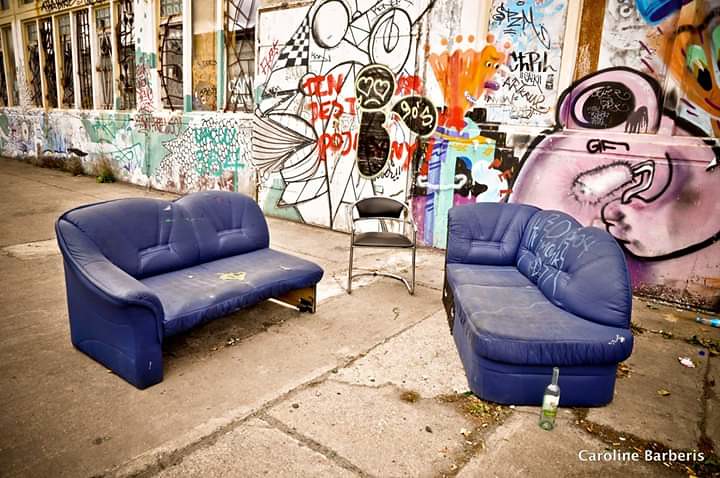This photograph captures a gritty urban scene, possibly in a back alley or slum area. The focal point is a pair of worn-out blue sofas, facing each other on a concrete walkway divided into square-like sections. The sofa on the right exhibits some graffiti and is exposing its foam interior, indicating prolonged exposure to the elements. A small black metal chair sits directly between the sofas, creating a makeshift seating arrangement. An opened wine bottle lies beside the right sofa.

In the background, a large wall, predominantly white but covered in vibrant graffiti, stretches across the image. On the bottom right-hand corner of this wall, a large pink creature with a massive black eyeball and an outstretched arm holding a paint roller stands out. Adjacent to this creature, a smaller black silhouette with heart-shaped eyes and a sad expression has a speech bubble saying "SOS". The wall also bears multiple other colorful designs and illegible tags, contributing to the overall eclectic aesthetic. Additionally, on the left side, several broken windows adorned with more tags further emphasize the setting's urban decay. The name "Caroline Barberis" is visible in the bottom right-hand corner of the image.